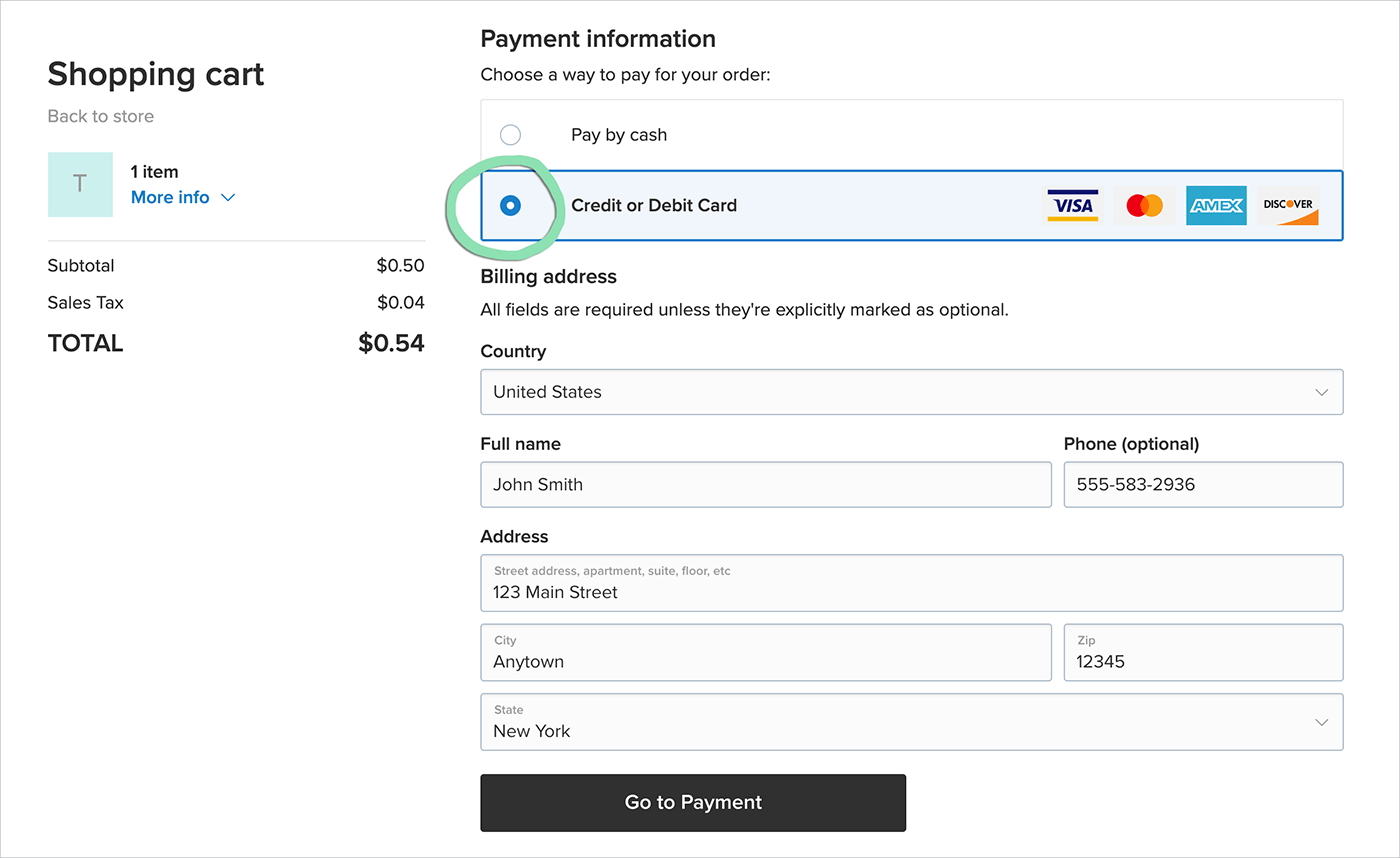This image is a screenshot of an online checkout page focusing on payment and billing information. 

At the top middle, the header reads "Payment Information," followed by the instruction "Choose a way to pay for your order." Beneath this, there are two options displayed in a rectangular box with two columns. The first column offers the option to "Pay by cash," indicated by a bubble to its left. The second column presents "Credit card or debit card," also with a bubble to its left. The bubble next to the credit/debit card option is blue and circled in green, suggesting it has been selected.

On the far right of this section, four familiar payment logos are displayed: Visa, MasterCard, Amex, and Discover.

In the top left corner, "Shopping Cart" is prominently displayed. Below this are several details: "Back to store," a letter "T," "1 item," and "more info" with a downward pointing arrow. Following this, cost breakdowns are listed: "Subtotal" is 50 cents, "Sales tax" is 4 cents, and "Total" is 54 cents. 

To the right of the screen, the section labeled "Billing Address" specifies that all fields are required unless marked as optional. The form includes fields for country, full name, and address.